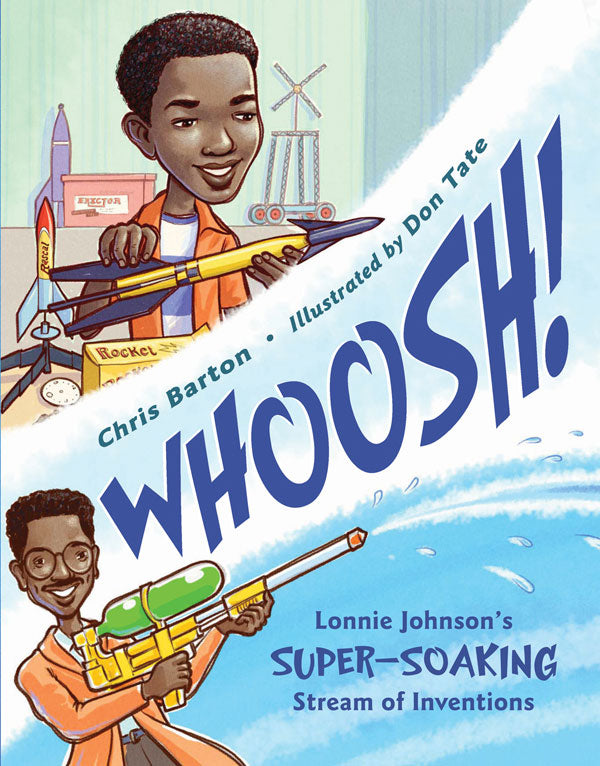The image is the cover of a book titled "Lonnie Johnson's Super-Soaking Stream of Inventions," with the text in blue located at the bottom right. In the foreground, there is a cartoon depiction of Lonnie Johnson, a Black man wearing glasses, smiling as he operates a Super Soaker. The Super Soaker features a green tube filled with water, a yellow and gray body, and a red tip. Lonnie is dressed in an orange suit jacket and gray pants, complemented by a blue belt.

In the upper part of the image, a boy with short brown hair is holding a toy rocket pointing to the right. He wears an orange shirt over a white and purple striped shirt. There are additional rockets and a box labeled "rockets" to his left, and another box in the background marked "Erector," with part of an Erector set visible. The background is blue, giving a vibrant feel to the illustration.

Above Lonnie Johnson's illustration, at the bottom, the cover also features the text "Chris Barton illustrated by Don Tate" and a large "WHOOOSH" to convey the dynamic action of the Super Soaker, with water squirting out.